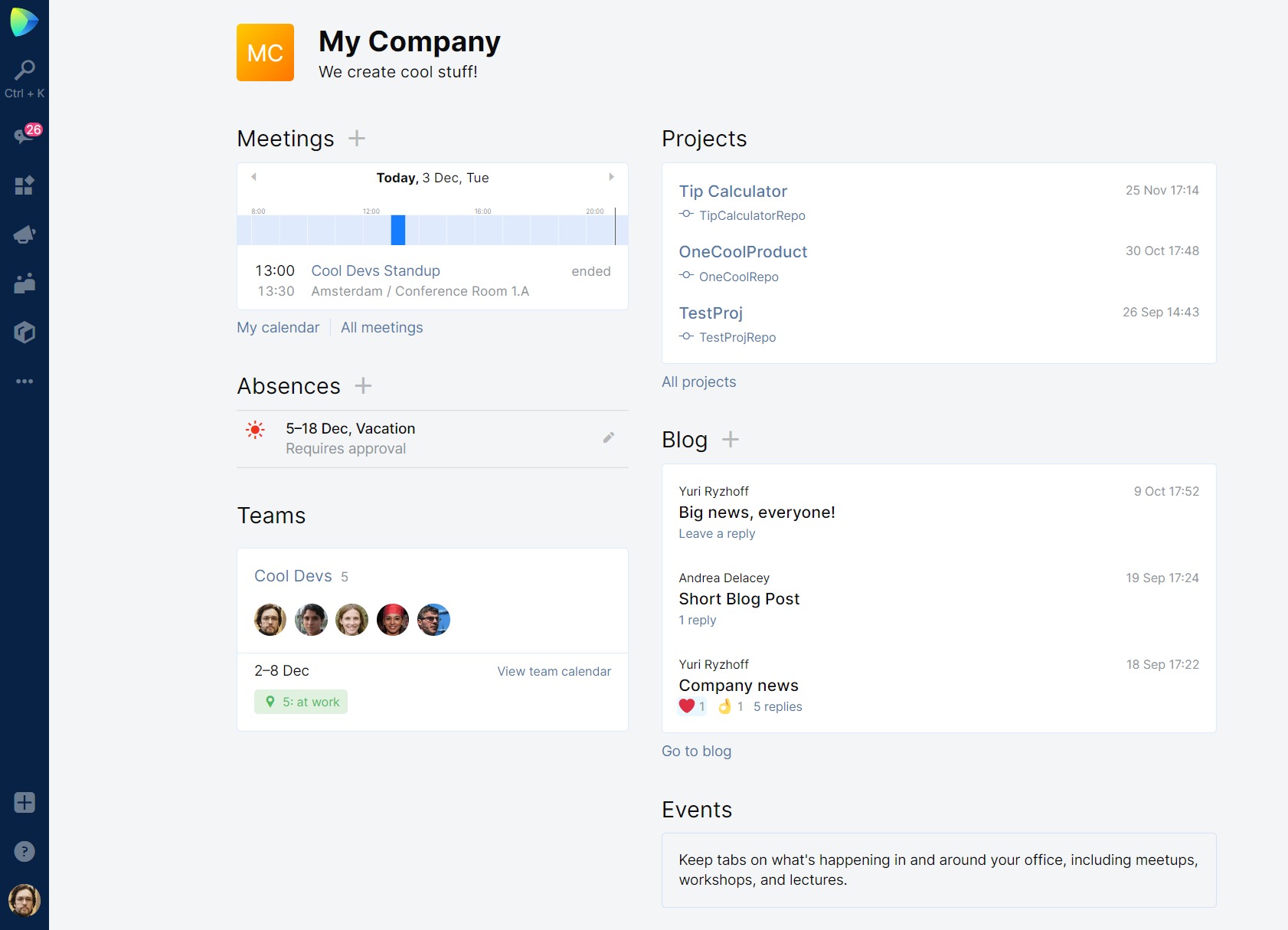This is a detailed screenshot of a website or application interface. On the left side, a dark blue vertical toolbar spans from top to bottom. At the top of the toolbar, there's a logo. Directly beneath it is a magnifying glass icon labeled "Control K." Below that, there are five different category icons arranged vertically. Further down, three dots indicate additional options. Near the bottom, there's a gray box with a cross inside, followed by a circle containing a question mark, and finally, at the very bottom, a circle with a user’s profile picture.

In the main body of the interface, at the top, there is a prominent yellow box labeled "MC," likely standing for "My Company," with some introductory text beneath it. Below this, the interface is divided into several sections:

1. **Meetings:** This section features a schedule displayed on a time bar.
2. **Absences:** A section with text pertaining to absences.
3. **Teams:** This section contains a white box labeled "Cool Devs," accompanied by circular profile pictures of team members and a date range reference, "2 to 8 DEC."

On the right-hand side, the interface includes additional sections:

1. **Projects:** This section has a white box listing various project names.
2. **Blog:** This area contains another white box with the names of different blog posts alongside their respective dates.
3. **Events:** The final section at the bottom includes a category for events followed by descriptive text.

The layout is organized and provides a comprehensive overview of meetings, absences, team information, projects, blog posts, and events, ensuring users can navigate and access information efficiently.